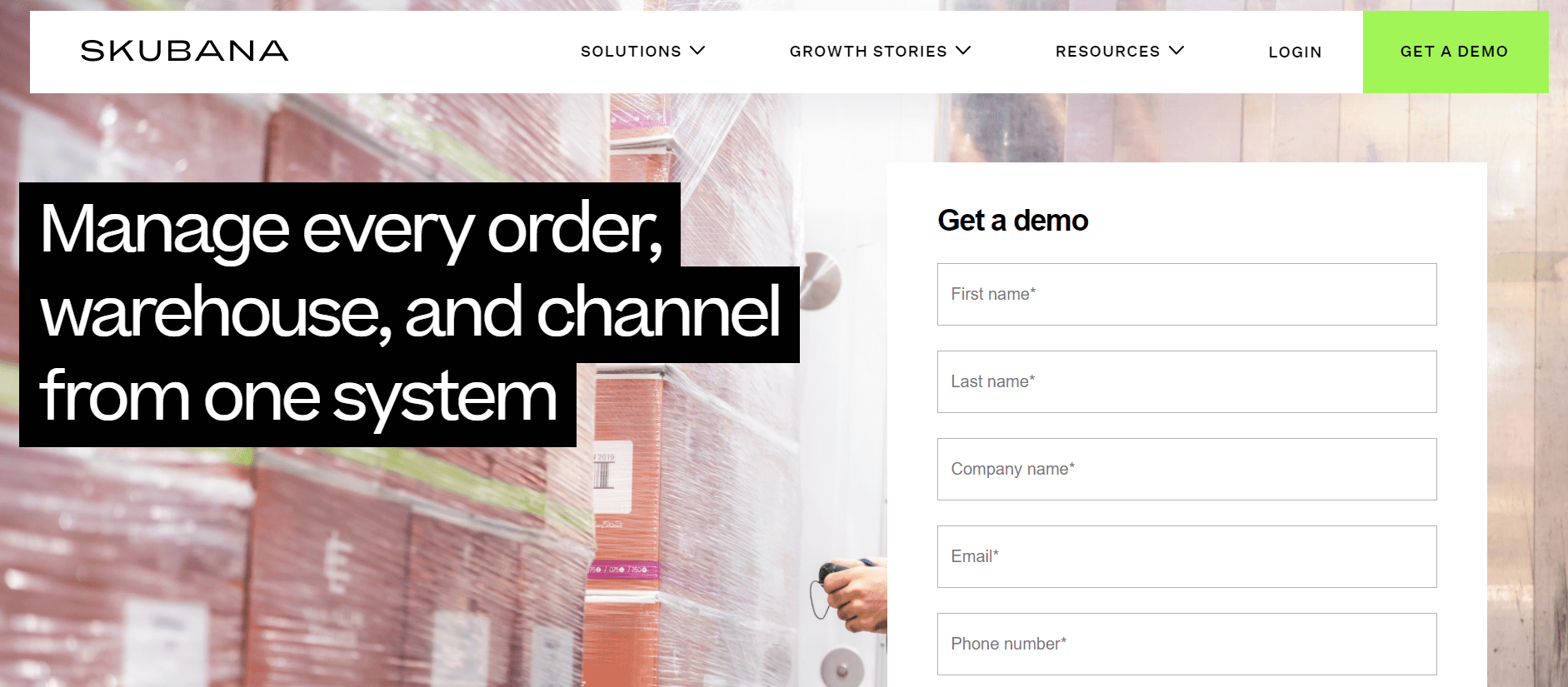The image captures a web page showcasing the Skubana platform. The top section features a white navigation bar with the Skubana logo on the far left, followed by drop-down menus labeled "Solutions," "Growth Stories," and "Resources." On the far right of this bar, there are two buttons: a white "Log In" button and a green "Get a Demo" button.

Beneath the navigation bar and the Skubana name, there's a prominent white text that reads, "Manage every order, warehouse, and channel from one system." This text is set against a black background that highlights each word individually.

To the right of this text, there's a white rectangle partially cut off at the bottom, containing fields for a demo request. The form fields include placeholders for the first name, last name, company name, email, and phone number.

The main background of the page appears somewhat abstract, possibly depicting stacked red boxes with a bright light illuminating them. A distinctive element within this background is a person's hand extending into the frame.